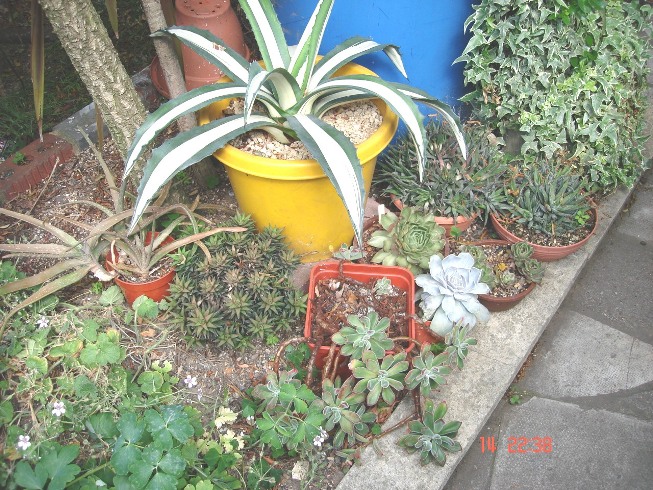In the image, a garden scene is captured featuring a variety of potted plants situated within a flowerbed. The flowerbed, raised and built between two curbs, showcases an assortment of different flowerpots, predominantly orange with one bright yellow pot standing out. This yellow pot contains a plant with green edges and white-centered leaves, which are large and drape over the sides of the pot. Adjacent to this pot is a smaller plant with circular, small green leaves. Scattered throughout the flowerbed are other potted plants with leaves of varying sizes, some in terracotta pots. A blue 50-gallon drum, possibly a rain barrel, is placed behind the yellow pot. The surrounding garden includes a stone walkway to the right of the flowerbed and a brick curb with grass on the opposite side. Also present is a small tree, visible mostly through its trunk. At the bottom of the image, a time stamp reads "14-22-38."